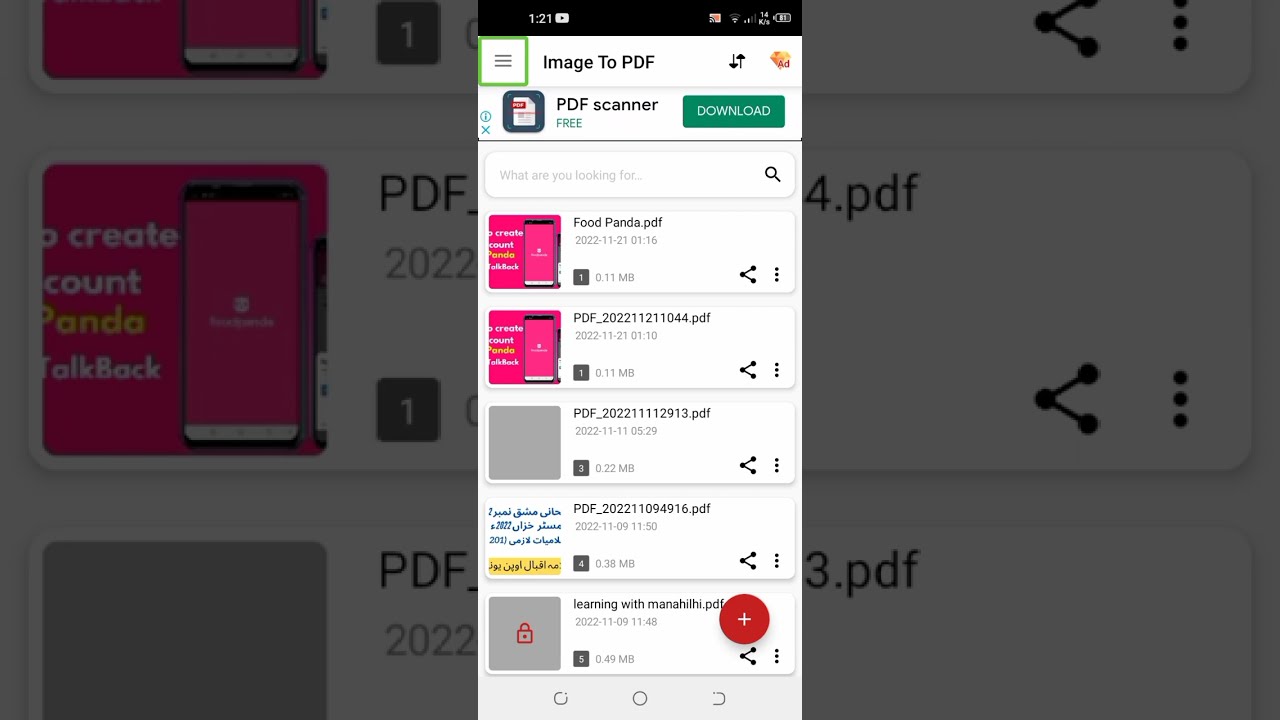This image is a composite screenshot from a smartphone, divided into three sections with the center showing the main content, and the left and right sections partially zoomed in and darkened. The main section of the image displays a mobile app titled "Image to PDF" that is designed for converting images to PDF files. At the top of the screen, indicators show the phone's battery level and Wi-Fi signal on the right, and the time (1:21) alongside a YouTube logo on the left.

Beneath the app's title, there is an advertisement for a PDF scanner marked by the word "Download" on a green button. Below this ad is a search bar with the prompt "What are you looking for?" and a magnifying glass icon. The main content area lists several PDF files with their names and sizes. The files are:

1. "foodpanda.pdf" (0.11 MB)
2. "pdf_2022112044.pdf" (0.22 MB)
3. "pdf_202211112913.pdf" (0.38 MB)
4. "pdf_202211094916.pdf" (0.49 MB)
5. "learningwithmanahillhigh.pdf" (size not explicitly stated)

At the bottom right, a red circle with a white plus symbol suggests the option to add more files. The overall layout features a clean, white background and typical Android navigation buttons at the bottom.